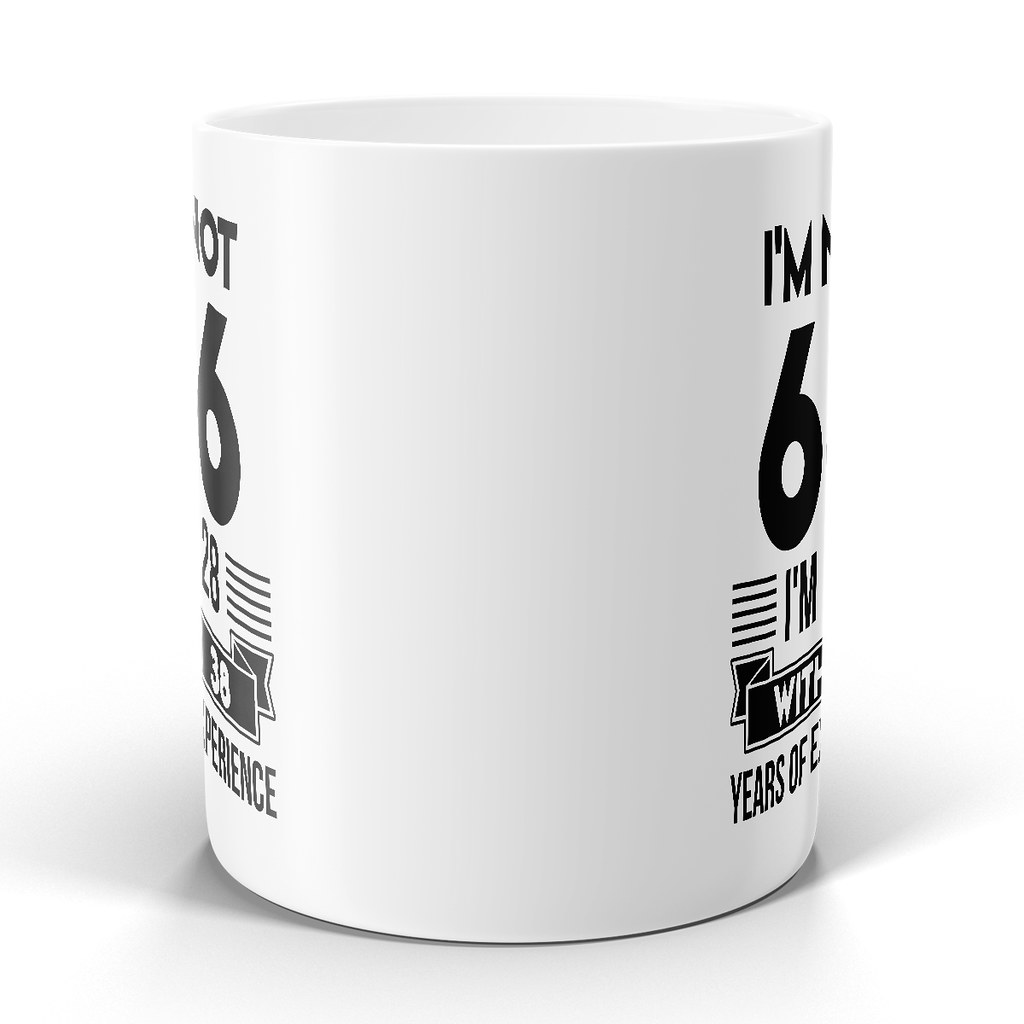This image showcases a high-quality white mug, presumably made from China, viewed from the side opposite the handle. Although we can't directly see the handle, the mug's design and size suggest its presence. The mug features a fancy black banner design with black lettering. The text is partially visible due to the angle, revealing phrases like "I'm," "6," "I'm with," and "years of experience." Piecing the clues together, the full message likely reads: "I'm not 66, I'm 28 with 38 years of experience." This humorous and somewhat tacky design implies it was a gift for someone's 66th birthday.